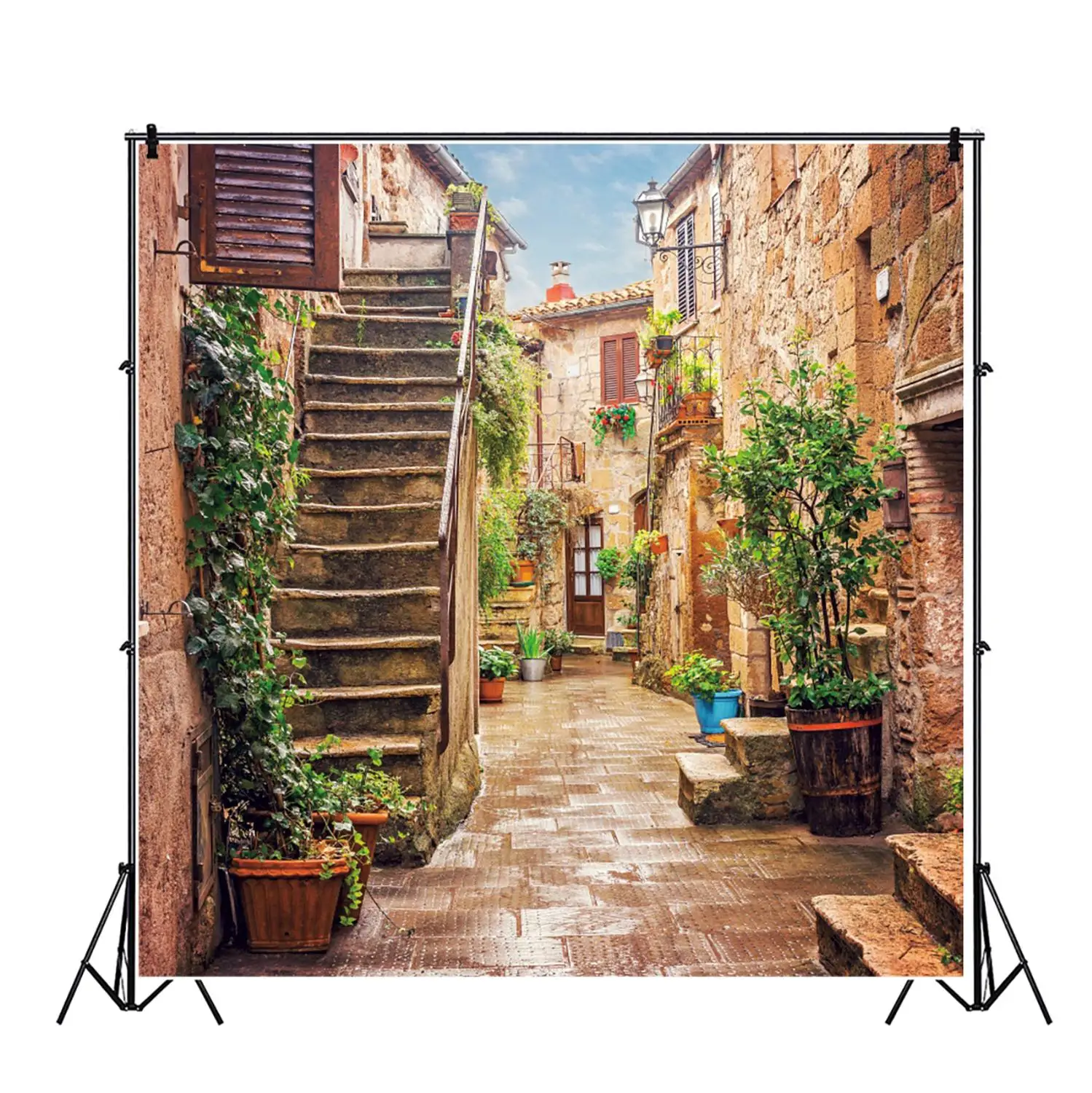The image, reminiscent of a painting, captures a quaint alleyway in a small town in southern Italy. It features old, brick buildings with wooden windows that open outwards. Narrow stone staircases and cobblestone paths add to the rustic charm. Planters with lush green plants and vines line the road, growing against the weathered walls. The sky above is blue with a few clouds, suggesting a recent rain shower. This scenic depiction is displayed as a photographic backdrop, mounted on two tripods with black clips holding a horizontal pole for stability. The backdrop creates an immersive scene, as if standing in the middle of the alley, facing the charmingly decayed buildings.